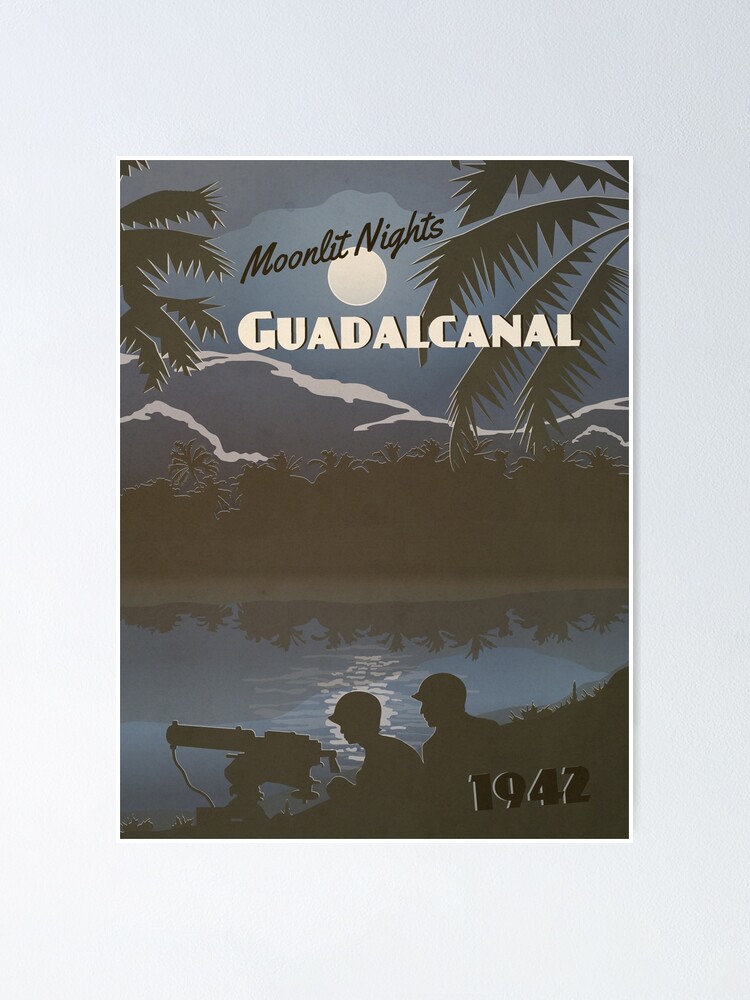This is a striking poster set against a white framed border, featuring an evocative scene rendered in dark blue, black, and white tones. Dominating the top portion of the poster, the bold black text "Moonlit Nights" is accompanied by a large, central moon. Just below, the name "Guadalcanal" stands out in white capital letters. The middle section of the artwork showcases a serene body of water, mirroring a dense row of palm trees and a mountain range beyond, both depicted as dark silhouettes with a hint of reflective blue tones. To the left and right edges, palm leaves are visible, partially extending into the scene. Central to this imagery, two silhouettes of helmeted soldiers crouch near the ground with a machine gun pointed leftward, adding a stark, poignant touch to the tranquil landscape. Positioned at an upward angle in the bottom right corner, the bold black date "1942" marks the historic significance of the piece.